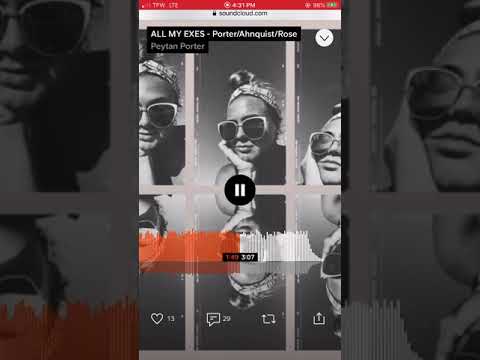A black-and-white image portrays a woman wearing sunglasses and a bandana, leaning on her hand pensively. The focal point is her face, while the background and edges feature additional close-up snippets of her expressions. On the interface, it's 4:31 p.m. on SoundCloud, displaying a track titled "Calm All My Exes" by Porter and Quiz/Rose Paste. The track is paused at the one-minute mark out of a total of three minutes, and it has garnered 13 likes and 29 comments. Bright interface elements, such as a refresh button and an upload button, are also present. An orange progress bar indicates the track is halfway played, with the remaining portion still white.